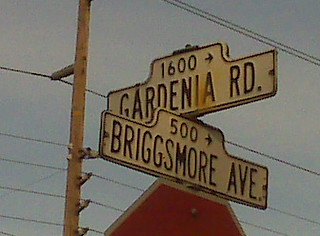In this photograph, there are two distinct street signs indicating an intersection. The first sign, featuring white lettering on a black background, marks "Gardenia Road." It has a rectangular shape with a slight protrusion at the top center, displaying the number "1600" and an arrow pointing to the right. Below it, running in a perpendicular direction, is a similar sign for "Briggsmore Ave." This sign also features white lettering on a black background, with the top center indicating "500" and an arrow pointing to the right. The image suggests it is located at the intersection of Gardenia Road and Briggsmore Avenue. Additionally, the partial top portion of an octagonal stop sign is visible beneath the Briggsmore Ave sign, indicating the presence of a stop sign at the intersection. The signs stand out sharply against their surroundings, helping to navigate the meeting point of these two roadways.